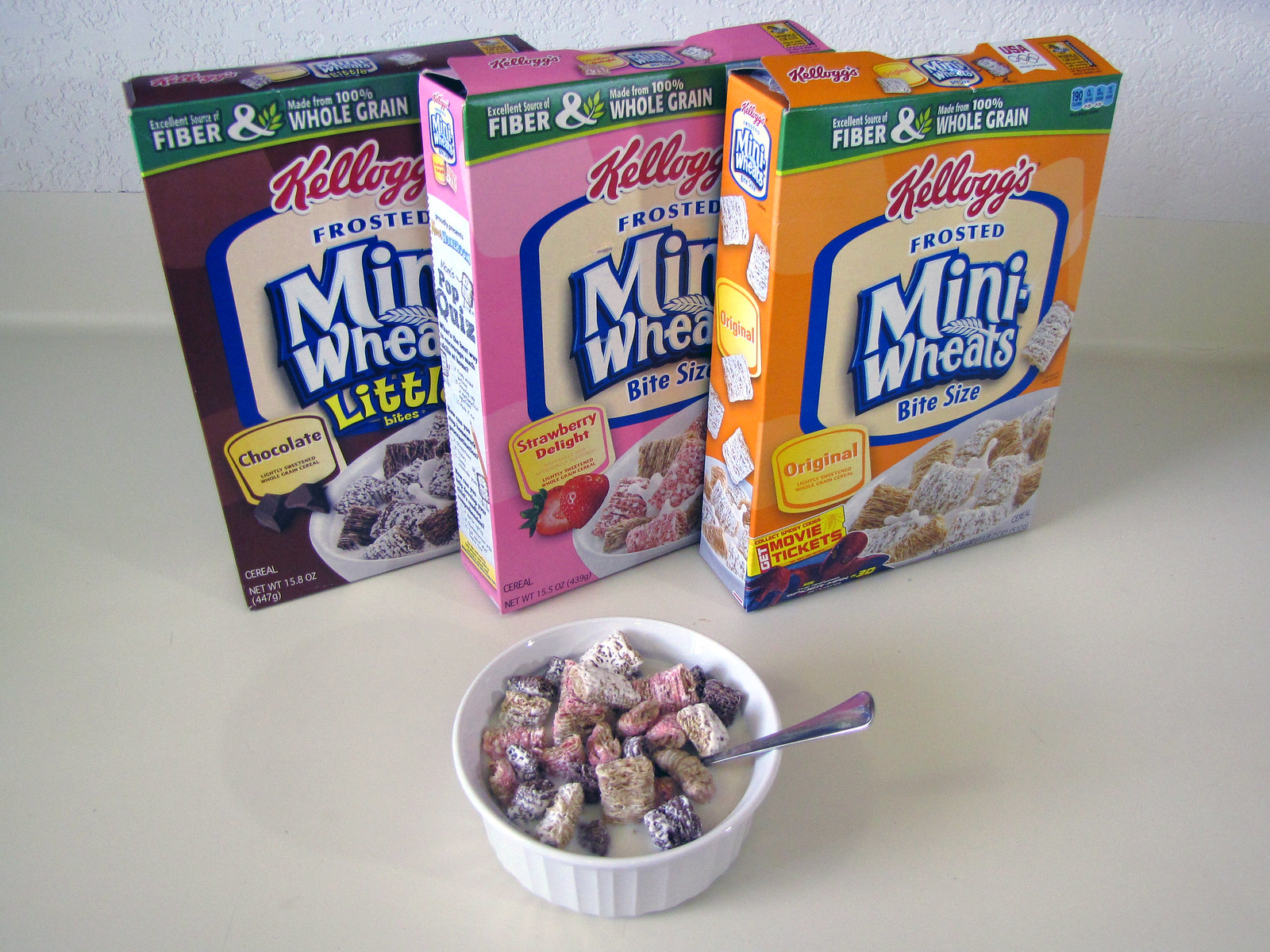This image portrays a detailed scene laid out on a cream-colored counter with a slight lip that rises against a textured white wall. At the forefront, there is a white, slightly fluted bowl with a smooth rim, containing a colorful mixture of mini wheat cereal pieces in shades of pink, blue, and their natural tone, suggesting the presence of multiple flavors. A silver teaspoon is placed in the bowl on the right side. The bowl is positioned in front of three distinctly colored boxes of Kellogg's Frosted Mini-Wheats. The box furthest to the left and slightly behind is the chocolate-flavored variant in a brown box, labeled "Kellogg's Frosted Mini-Wheats Little Bites." The middle box, pink and labeled "Frosted Mini-Wheats Bite Size Strawberry Delight," stands out next. The third and closest box on the right is the original flavor in an orange box, also marked "Frosted Mini-Wheats Bite Size" featuring an advertisement for movie tickets at the bottom. Each box prominently highlights that the cereal is made with 100% whole grain and provides fiber. The assortment in the bowl reflects a blend of all three cereal flavors, visually inviting and well-arranged, positioned strategically against the minimalist white backdrop.